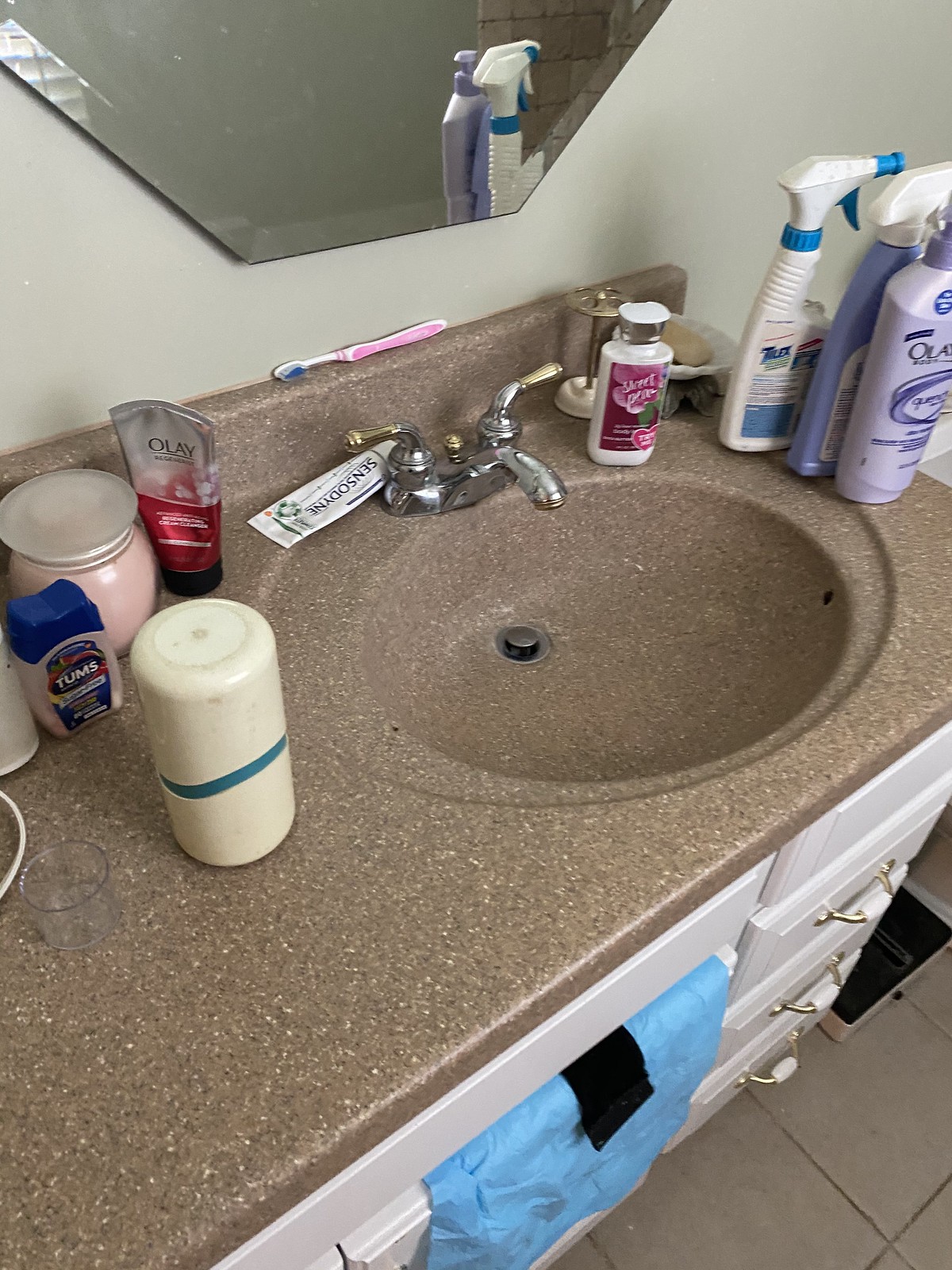A bathroom vanity is prominently featured in this image. The countertop of the vanity is a medium brown with scattered white speckles, exuding a refined elegance. The matching backsplash seamlessly blends with the countertop, and both the sink and backsplash are constructed from the same speckled material. A partial mirror is visible above the backsplash, contributing to the sense of space.

A chrome faucet with gold-accented handles is mounted on the countertop. Various toiletries are neatly arranged on the surface: a toothbrush placed on the backsplash, a bottle of Tums, a tube of Olay skincare product, Sensodyne toothpaste, some lotion, Tilex cleaner, Olay bath wash, and another unidentified cleaning product.

The vanity itself is made of wood, featuring drawers and cabinet doors beneath the sink. Draped over one of the cabinet doors is a piece of blue paper with a black item resting on it. The floor is tiled, adding to the room's polished look, and a heat register is situated near the base of the vanity, blending functionality with the bathroom’s aesthetic.